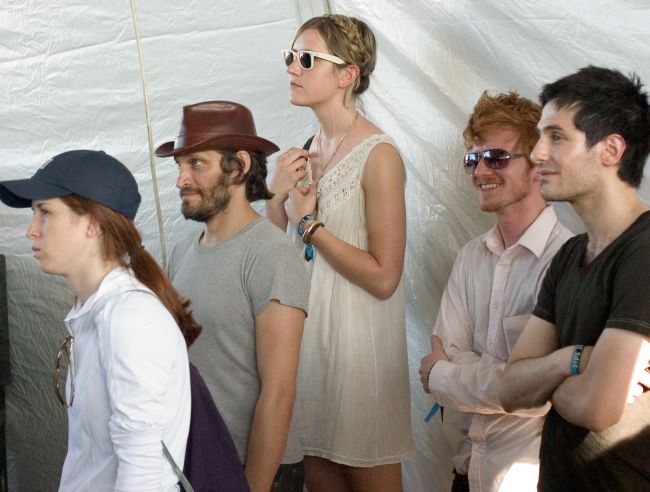In the photograph, five individuals are all gazing towards the left, set against a heavily wrinkled white fabric-like background. On the far left, a woman with long brown hair tied into a ponytail wears a blue baseball cap and a white button-up shirt, with glasses hanging from her collar and a purple backpack with gray straps. Next to her is a man in a short-sleeve gray t-shirt, sporting a beard and short-cut hair, and wearing a rounded brown fedora. At the center of the image is a taller woman in a sleeveless white sundress with white-rimmed, black-legged glasses. Her hair is styled up, creating a crown-like effect, and she adorns multiple bracelets on her wrist. To her right, a man wearing black pants and a partially unbuttoned white shirt stands with his arms crossed in front of him. Both he and the next person, on the far right, who is also wearing a white button-up shirt with the top button undone and has his arms similarly positioned, are looking off to the left.